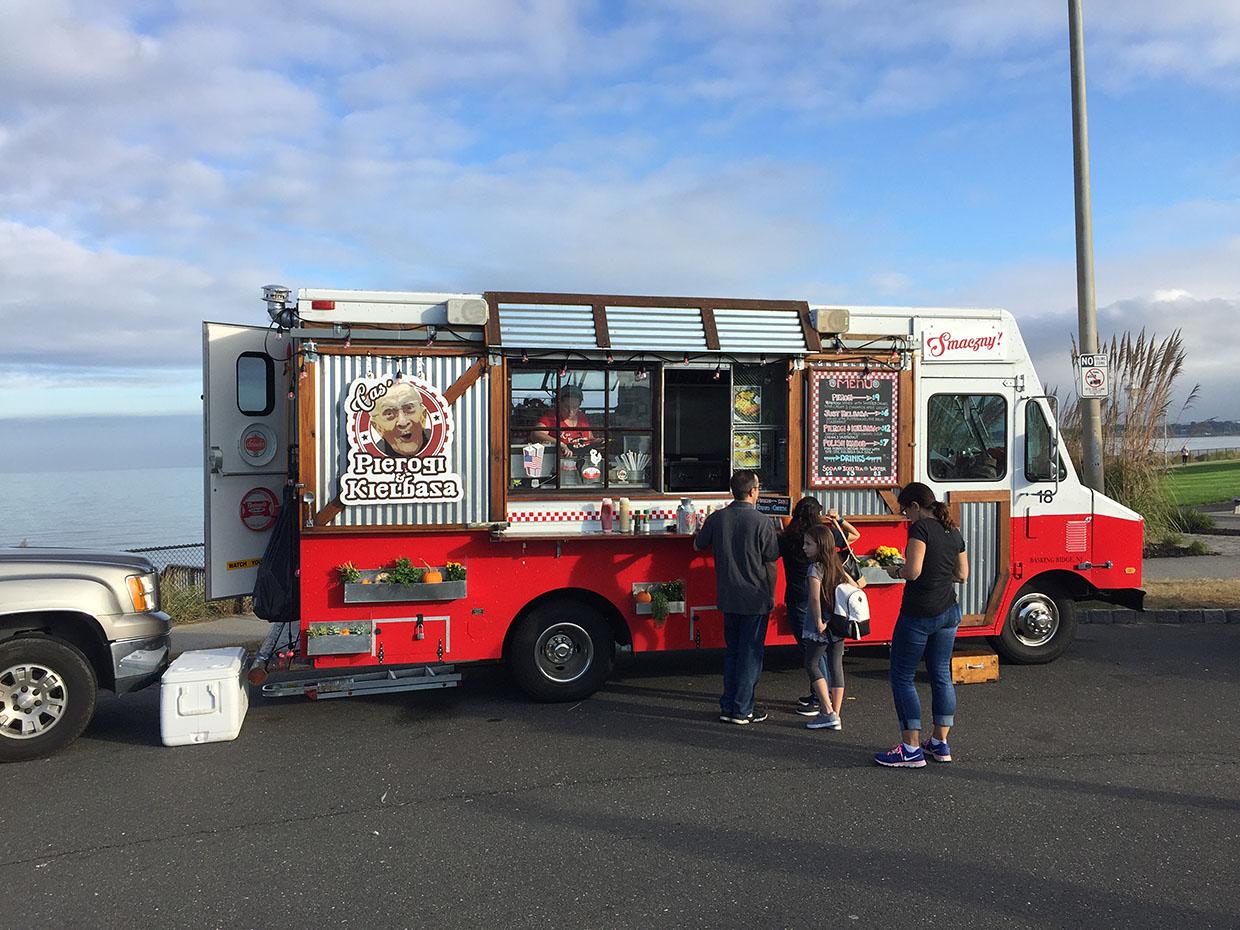This vivid photograph captures a bustling scene centered around a large food truck, prominently situated on a gray asphalt road. The food truck, marked by its vibrant red bottom and clean white top, features a large serving window bustling with activity. A woman dressed in red is seen serving eager customers, with three to four individuals waiting in line for their orders.

Bright signage on the left side of the truck boldly announces "Cass's Pierogi and Kielbasa," accompanied by a logo depicting an old man’s face. Notably, a "No Parking" sign, humorously including "No Food Trucks," stands defiantly in the foreground, adding a touch of irony to the scene.

To the right of the truck, the setting transitions into a quaint park area, with a small sidewalk leading to a sprawling green space and a large, peaceful body of water beyond. The backdrop is completed by a serene blue sky filled with scattered white clouds. Behind the food truck, a partial view of a gray car and a white cooler box can be seen, adding to the sense of a lively, community-oriented day. The overall ambiance suggests a beach town atmosphere, potentially attracting numerous visitors and creating a vivid scene of local life.